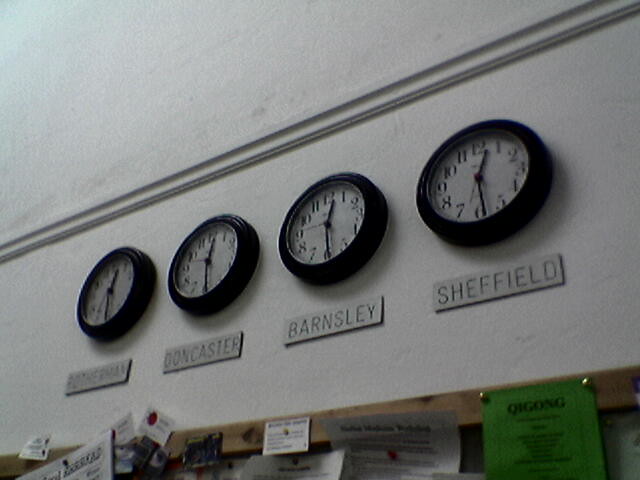The image depicts a white wall adorned with four uniformly styled clocks, each housed in a black case with a round border. The clocks feature white faces with black numerals and hands, all showing nearly the same time, approximately 12:29 or 12:30. Below each clock, there are metal nameplates with engravings that identify different locations: from left to right, these read Rotterdam, Doncaster, Barnsley, and Sheffield. Beneath the nameplates, a light beige wooden bulletin board is attached to the wall, holding an assortment of notes and cards. These assorted papers, including one green piece and several white ones with black or blue writing, are pinned down with gold thumbtacks.